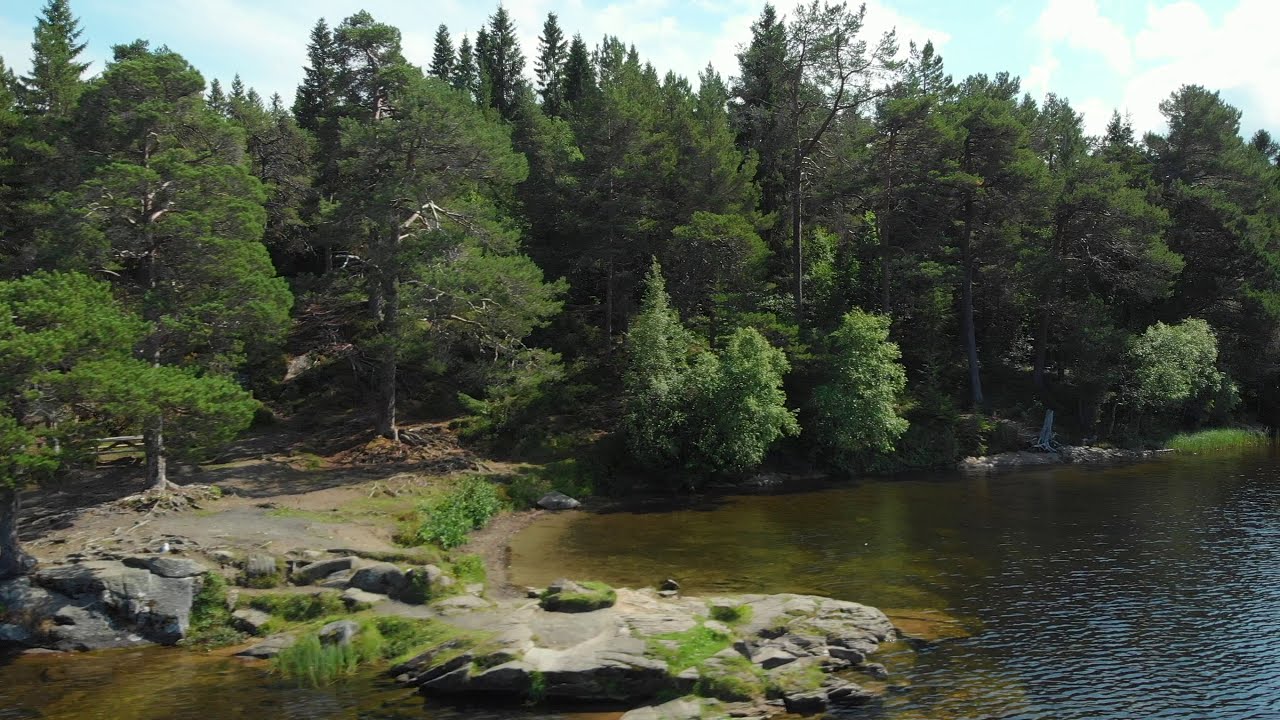The image captures a serene natural landscape featuring a lake with calm, rippling water that takes on a greenish algae hue. The lake is bordered on the right by a rock platform topped with grass, which transitions into a dirt bank as it ascends. This dirt area is edged by a thick forest, teeming with lush, green trees that include both evergreens and deciduous varieties. The dense canopy is impenetrable to the eye, creating a solid green backdrop. Above the trees, the vibrant blue sky is scattered with fluffy white clouds that reflect sunlight, enhancing the tranquil atmosphere. Light also dances off the lake's surface, especially in the bottom right corner, while other areas lie in the shadow of the rolling hills covered by the forest. The entire scene exudes calm on a beautiful, seemingly warm and windless day, devoid of any human presence.